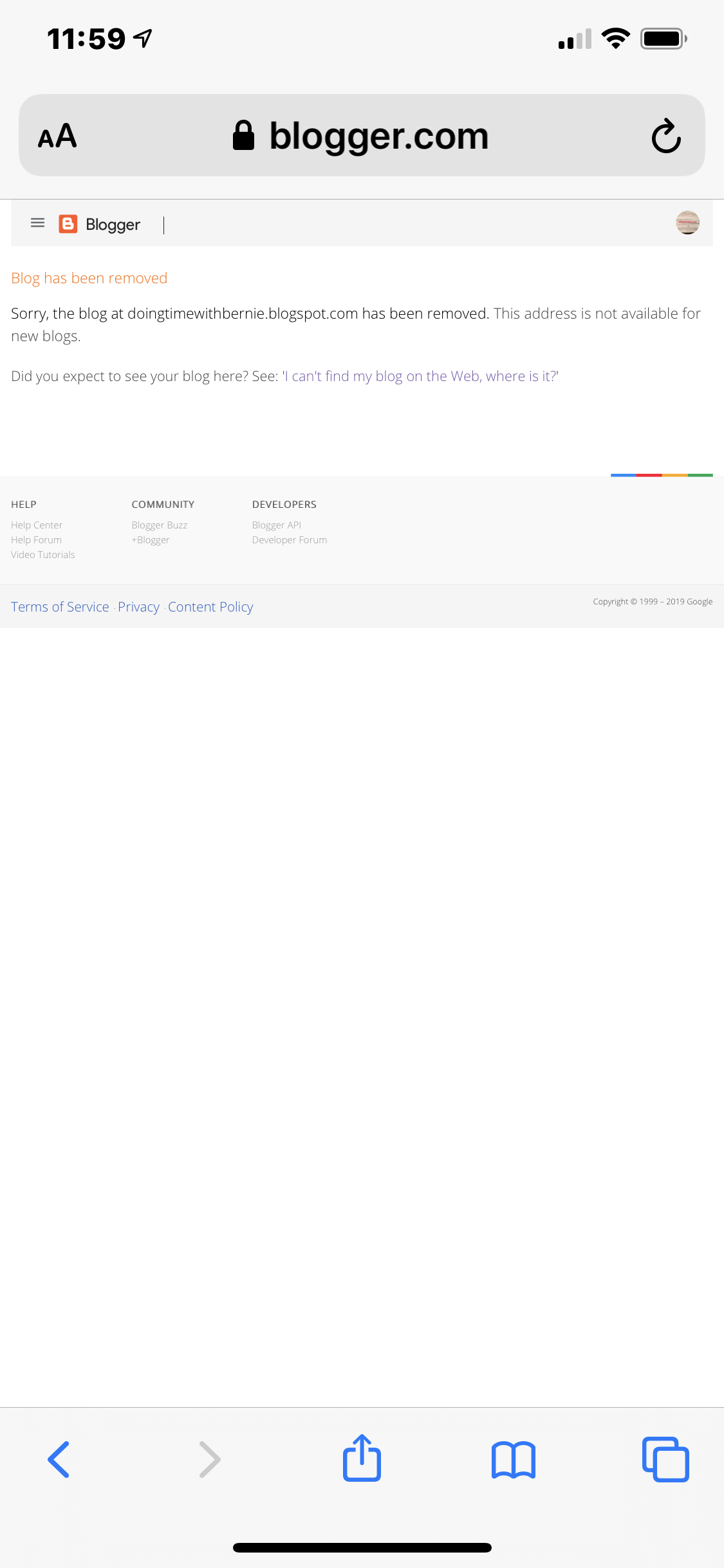A mobile screenshot captures a webpage on Blogger.com indicating a blog has been removed. At the top, the browser's search bar displays "blogger.com." Directly beneath it, a grey header bar features the Blogger logo on the left side. The main body of the webpage is stark white, with a prominent message in orange text on the top left that states, "Blog has been removed." Beneath this, a smaller black text message reads, "Sorry, the blog at doingtimewithbernie.blogspot.com has been removed. This address is not available for new blogs."

For users seeking assistance, a hyperlinked question appears: "Did you expect to see your blog here? See I can't find my blog on the web, where is it?" 

At the bottom, a grey footer bar is organized into three categories: Help, Community, and Developers, each with a vertical list of options. The phone's browser options are visible at the very bottom of the screenshot. To the left, there's a left-pointing arrow for going back; in the center, a send or share icon is displayed; to the right, there's a page view icon, and at the far right, a minimize windows icon.